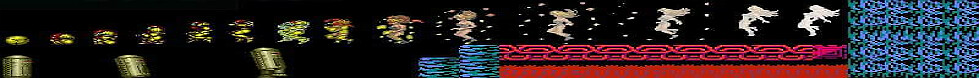This image is a still from a video game or digital artwork, captured in a highly elongated, banner-like format. The entire backdrop is a solid black, providing a striking contrast to the vibrant elements that populate the scene. 

Starting from the right, the image features blue and green shapes that may represent water, which transition into a red and gold area that forms an intricate pattern resembling the letter "A". This serves as a platform where characters, initially appearing as small yellow or gold dots, begin their transformation. These characters grow larger and more detailed as they move leftward across the image.

In the middle section, the yellow shapes evolve into a cream-colored body surrounded by dots, and on their journey, these forms are shown jumping and changing as if using a spring, with new clothing and hair arrangements appearing on the figures. Eventually, these characters become more spirit-like, floating with flowing hair and limbs extended, surrounded by three golden cylinders with intricate designs.

Towards the end of the strip, the image shifts again, featuring blue, pink, and purple patterns along the bottom, with the final section showcasing a green ball-like figure against the emptiness of the black background, marking the conclusion of this visual evolution. The image effectively captures the transformation of these characters in vivid detail, set against a minimalist yet dynamic backdrop.